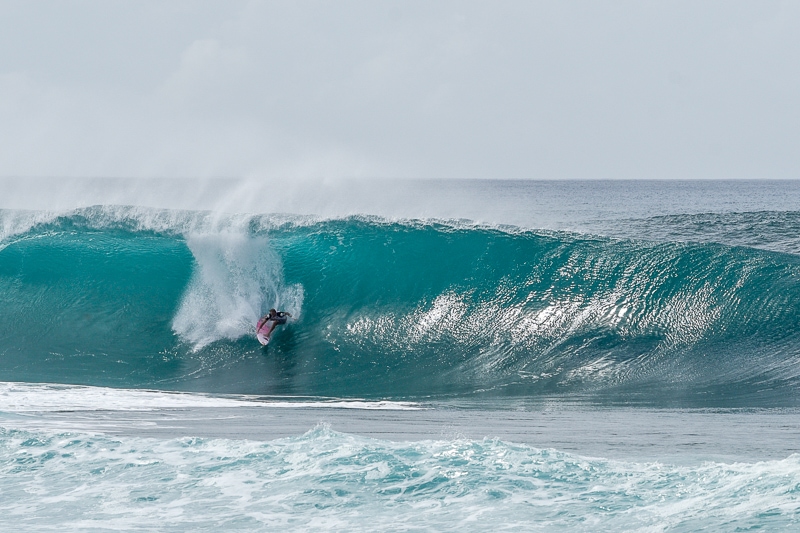This outdoor action photograph captures a striking image of a surfer catching a wave in the ocean. The sky above is a light, overcast gray, creating a muted backdrop that contrasts with the dynamic scene unfolding in the water. The focal point is a large, horizontal turquoise blue wave that is just beginning to crest but hasn't broken yet. On the left side of the wave, approximately two-thirds down from the top, a surfer in a black wetsuit rides a white surfboard with a muted pink back. The surfer is crouched, with their right arm hanging straight down and their left arm by their side, as the surfboard kicks up a dramatic spray of white water. This spray, visible along the left and back sides of the surfer, highlights the energy and motion of the scene. The foreground of the photo shows darker water topped with white foam, suggesting that the waves are moving towards the shore. Despite the gray sky, the photograph is well lit, capturing vivid details of the turbulent ocean and the powerful wave.